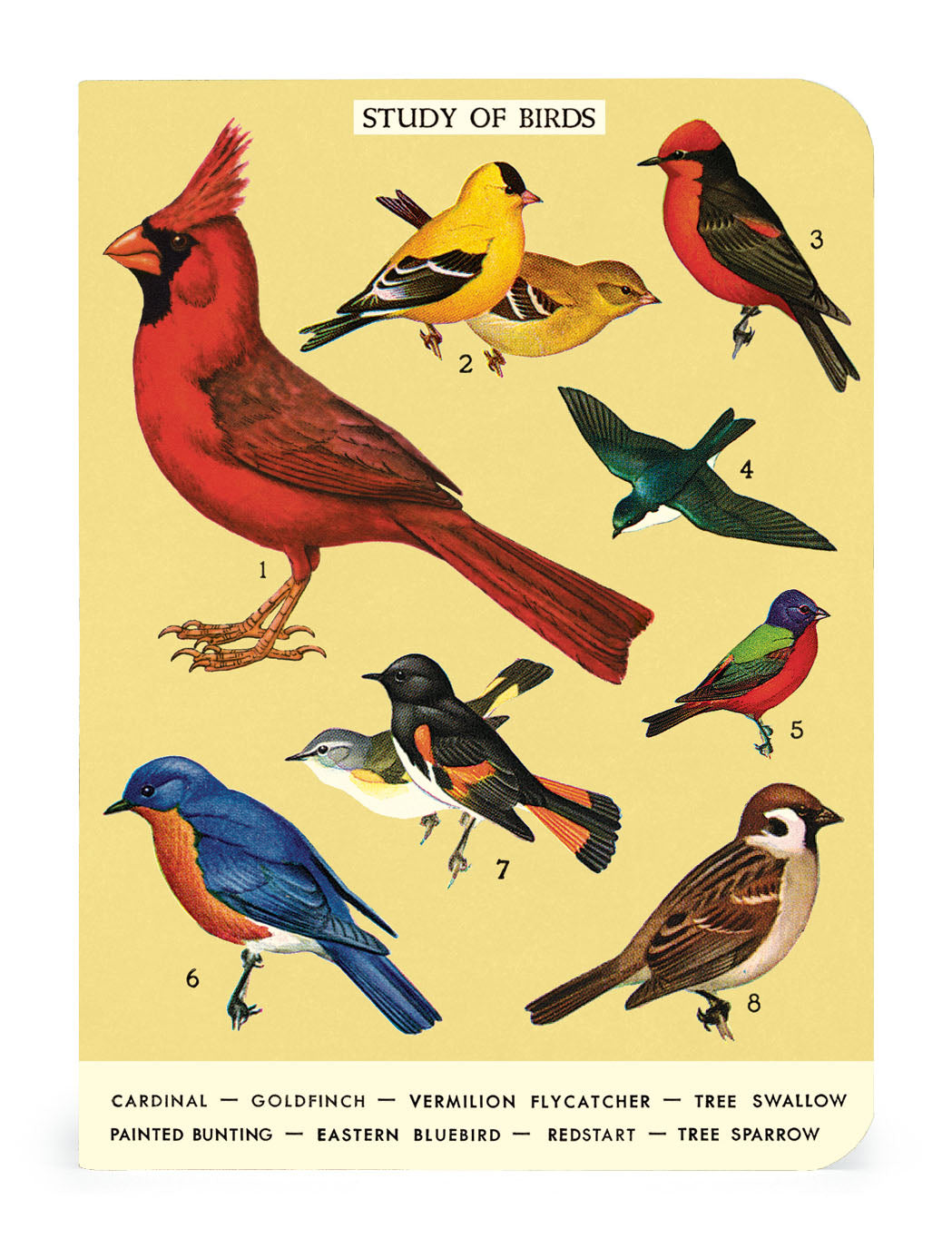This vintage-looking, square-shaped illustration with a pale yellow top and curved corners on the upper right and lower left features a detailed "Study of Birds" header in a small white rectangle. Numbered 1 through 8, the richly colored, albeit slightly faded, hand-drawn birds include a vibrant Cardinal, two striking yellow Goldfinches, a vivid red and black Vermilion Flycatcher, a greenish Tree Swallow in flight, a multicolored Painted Bunting, a brown and white bird, a black and gray species, and a blue-backed Eastern Bluebird with an orange belly. The bottom of the card lists the bird names in black text, though they don't directly correspond to each image. The meticulous artwork showcases a captivating array of avian diversity, emphasizing the artistic beauty of these varied species.